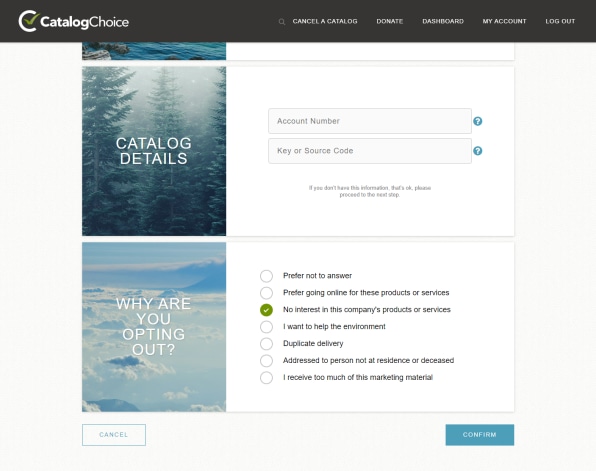The interface screen features a black header at the top and a sidebar on the left. The left sidebar displays a circular graphic resembling a partially completed circle, akin to a "C," with a check mark to the right of it. This area prominently displays the text "Catalog Choice" in white and gray letters. On the right side of the header, there are navigation options listed in white text: "Cancel a Catalog," "Donate," "Dashboard," "My Account," and "Log Out."

Beneath the header, to the left, is a picture captioned with "Catalog Details" in bold, white capital letters. The image depicts a foggy forest scene, with trees partially obscured by dense fog. Below this, there's another image resembling an aerial view from an airplane, showing a layer of clouds. This image is labeled with "Why are you opting out?" in white capital letters.

On the right side of the screen, there is a box labeled "Account Number" with a field for users to input their account details. Below this is another input field labeled "Key or Source Code," accompanied by a note stating, "If you don't have this information, that's okay, please proceed to the next step." Underneath these fields, there is a checkbox option labeled, "No interest in this company's products or services."